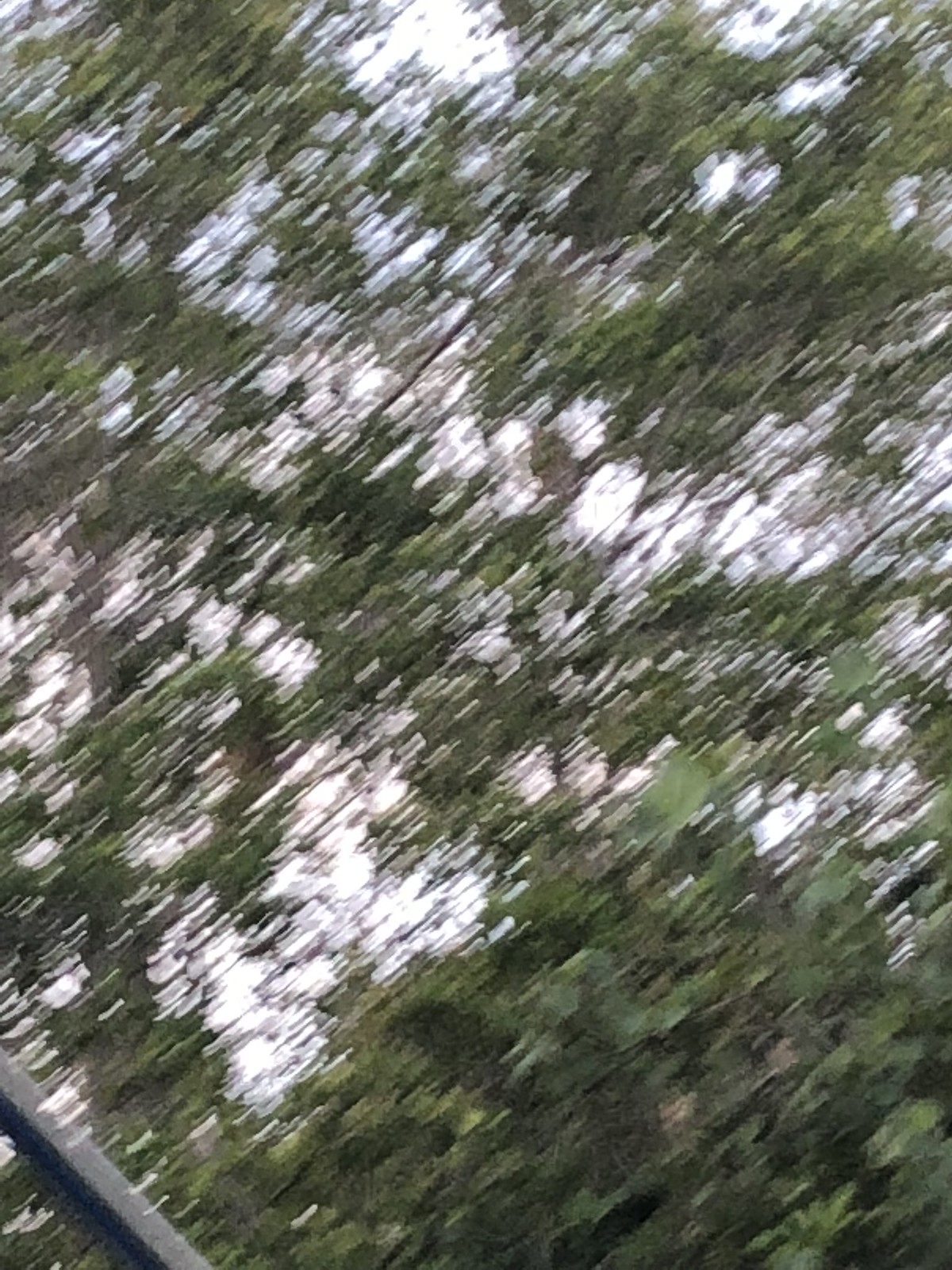This image appears to be a highly blurred photograph likely taken from the window of a moving car, capturing motion as it focuses on an area of dense greenery and trees. The trees, exhibiting a spectrum of light to dark green hues, appear smeared and out-of-focus, almost as if they are dripping, due to the motion. In the background, patches of clear blue sky interspersed with white clouds can be seen peeking through the foliage, adding to the dynamic feel. In the bottom left corner, a vague black line, possibly part of a car's window or an electrical wire, is visible, while the bottom right is dominated by more indistinct trees, absent of any visible sky.